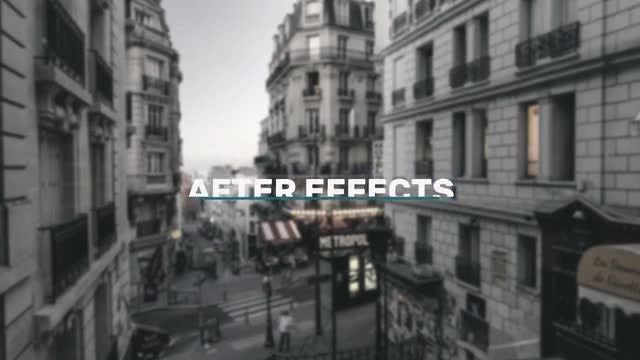This somewhat blurred black-and-white photograph captures a city street flanked by buildings, which appear to be constructed of either white or dull gray brick. In the center of the image, large white letters spell out "After Effects" with a blue line beneath them, though it is slightly misspelled as "E-F-F-F-C-T-S." The sky in the background appears dull and gray, contributing to the overall grayed-out ambiance of the image.

The buildings on each side of the street have distinctive white stone facades with black window sills, and some have little balconies extending from the windows. A notable detail is a yellow light glowing from one of the windows, casting a subtle illumination on the side of a building further back. Additionally, a maroon and white awning covers a stand near the sidewalk, adding a touch of color to the otherwise monochromatic scene.

A white crosswalk is clearly marked on the street, where several people can be seen, albeit faintly due to the increasing blur towards the background. In particular, one person is discernible wearing black pants, a white top, and brown hair, suggesting the image was taken from an elevated vantage point.